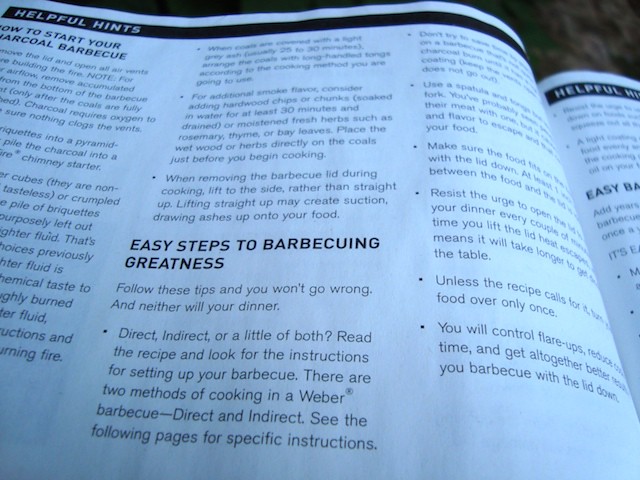In this detailed photograph, we see an open book, possibly a manual for a Weber charcoal grill or a cookbook. The primary focus is on the mostly visible left-hand page, with a tiny part of the right-hand page also in view. Dominating the top of the page is a black banner with bold, white capital letters stating "HELPFUL HINTS." Below, the left column is titled "How To Start Your Charcoal Barbecue," detailing necessary steps across a column and a half. Further down, a new section emerges in all caps: "EASY STEPS TO BARBECUING GREATNESS," offering practical tips to ensure successful barbecuing. The text in these sections is rendered in small black letters on the otherwise white page. The book rests on a dark wooden surface, enhancing the contrast and making the detailed instructions stand out.